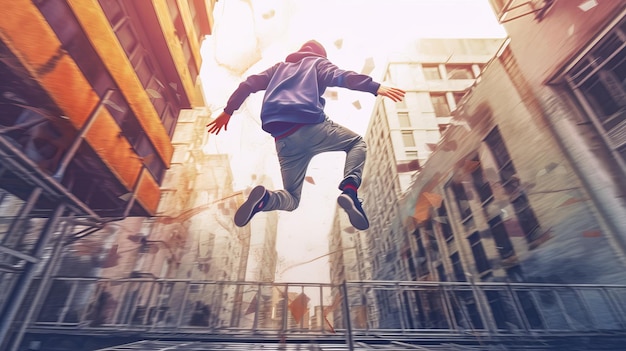In this captivating image, a person is captured mid-jump, soaring high into the sky. The person, seen from behind in a dynamic mid-air pose with their legs bent and arms splayed, is sporting a backwards baseball cap, a blueish-purple sweatshirt, light gray pants, and black tennis shoes. The backdrop features tall, cream-colored and brown buildings, with one distinct orange building on the left side, giving the impression of a city street scene. Shot from a low angle, the bright white sky dominates the background, while a horizontal metal railing, resembling a sideways ladder, spans across the bottom portion of the image, adding an interesting linear contrast to the verticality of the buildings and the energetic leap of the jumper.